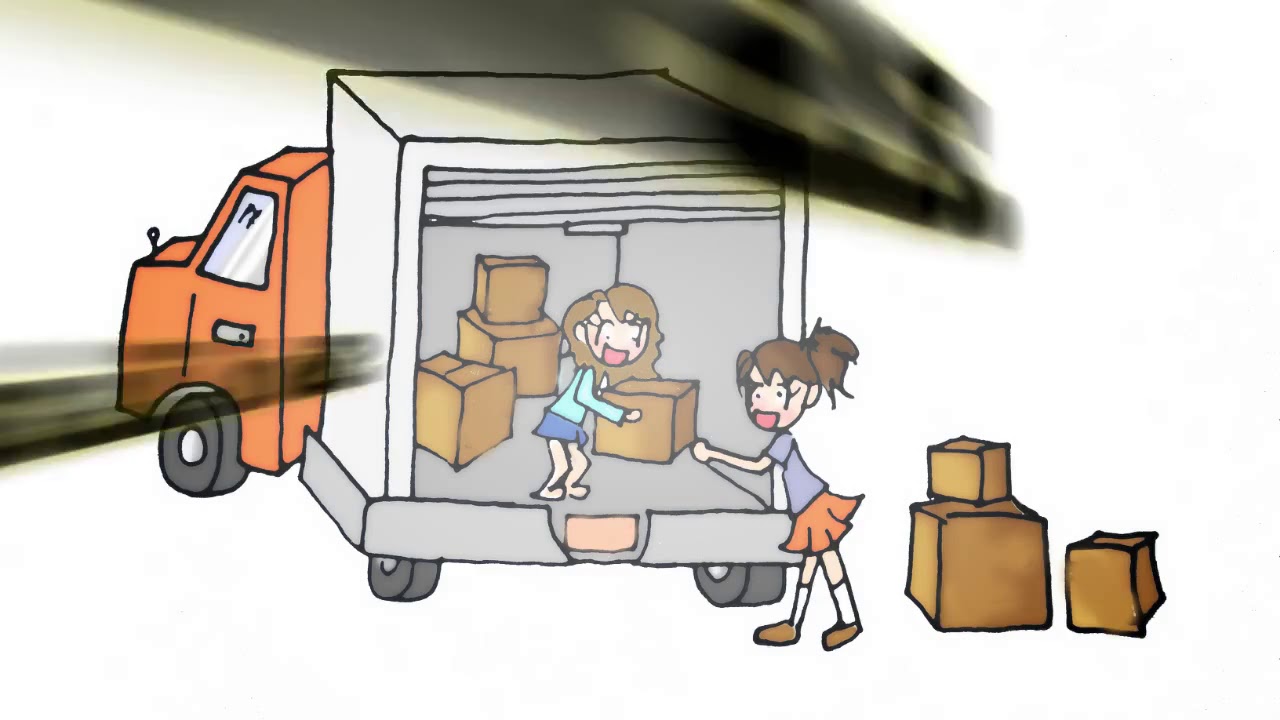A detailed cartoon drawing depicts two girls working together to unload a white box truck with an orange cab and black tires. The truck's cab, which includes a small grayish-white window, is directed towards the left, bending slightly away from the trailer. The back section of the truck is filled with neatly stacked brown boxes, creating a busy scene.

The girl inside the truck stands barefoot and holds a brown box. She has light brown hair and wears a light teal long-sleeved shirt with a blue dress. Opposite her, on the ground, is the second girl, identified by her brown hair pulled into a ponytail. She is dressed in a pink shirt, an orange skirt, white socks, and brown shoes. Both girls interestingly have their tongues sticking out, adding a playful touch to the scene.

The second girl's left arm is extended, ready to receive the box from her companion. Around the ground near her, three brown boxes are visibly arranged. Further detail in the image shows the back of the truck with the sliding door mechanism and a light orange rectangle that resembles a license plate positioned centrally below the open doorway. The backdrop also features two streams of black streaks with indistinct markings, one forming a letter "S" and the other the number "2," adding intriguing elements to the overall scene.